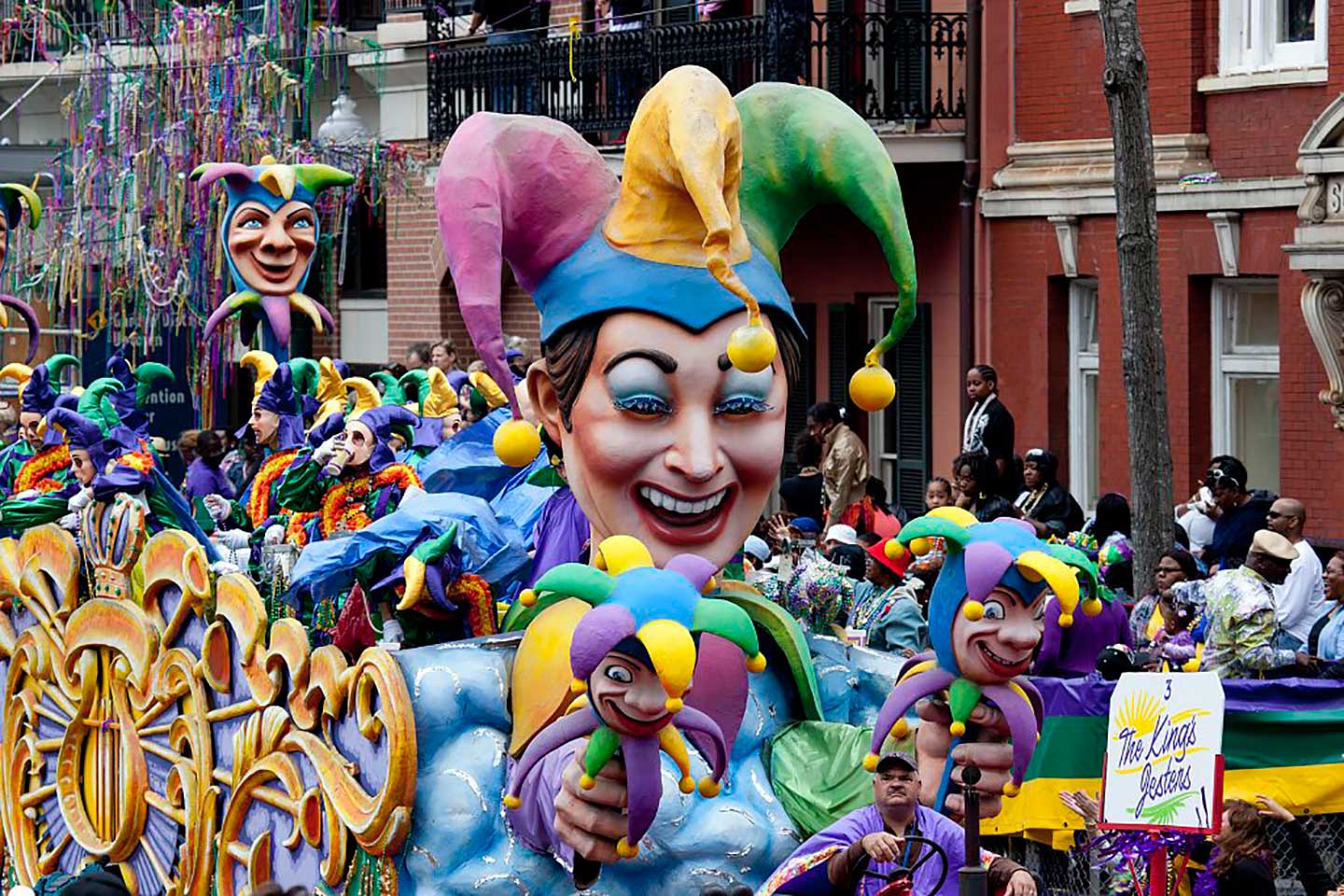The image depicts a vibrant Mardi Gras parade on a street lined with red brick buildings, typical of New Orleans architecture. These buildings showcase distinctive ironwork balconies festooned with colorful streamers and beads. In the foreground, a large, elaborate float features an oversized jester with a gigantic head adorned with a multicolored hat in purple, yellow, and green, complete with tassels or pom poms. This main jester is holding miniature jester figures in each hand. A sign near the float reads "The King's Jesters," underscoring the theme. Among the revelers, a man in a purple shirt, positioned at the bottom of the float with a steering wheel, appears to be driving it. The float is surrounded by costumed participants dressed in colorful jester outfits, with hues of purple, green, and yellow, often adorned with flowers around their necks. In the background, trees draped with bead necklaces add to the celebratory atmosphere, while numerous spectators line the sidewalks, eagerly watching and reaching towards the vibrant, intricately designed parade float.